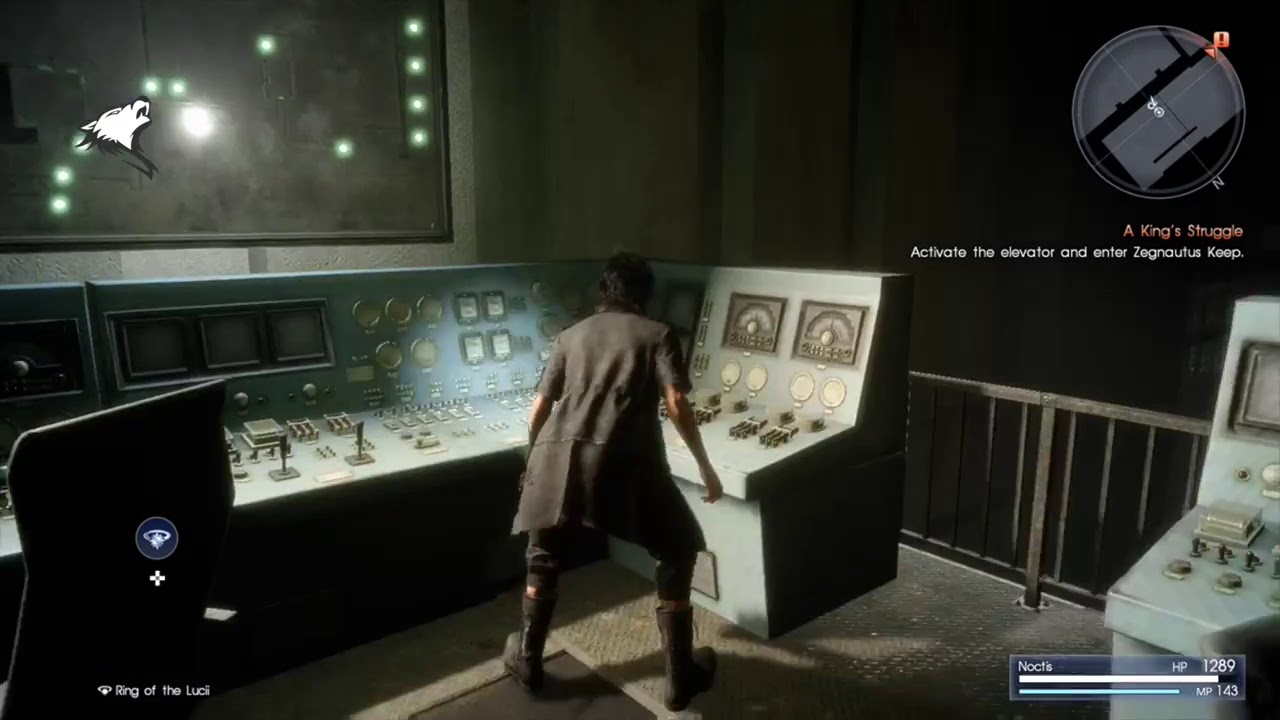The highly detailed, realistic video game screenshot features a man standing at a control panel in what appears to be a mission-driven environment. The character is clad in a black and gray trench coat-style outfit, black boots, and brown pants. In the background, illuminated by various control interfaces, there is a mission directive displayed with the text, "Activate the elevator and enter Zanginus Keep," under the overarching mission title, "A King's Struggle." The control panel in front of the character is equipped with numerous LEDs, dials, knobs, and screens, one of which displays a map with black dots and a radar in the upper right corner. The bottom left corner has the text "Ring of Lucci." Additional details include a monitor that shows a howling wolf face among green orbs and dots, and a numerical readout stating HP 1280. A black chair is positioned to the lower left of the panel, and a railing separates the control area from a wall with a window, adding to the immersive control center setup.